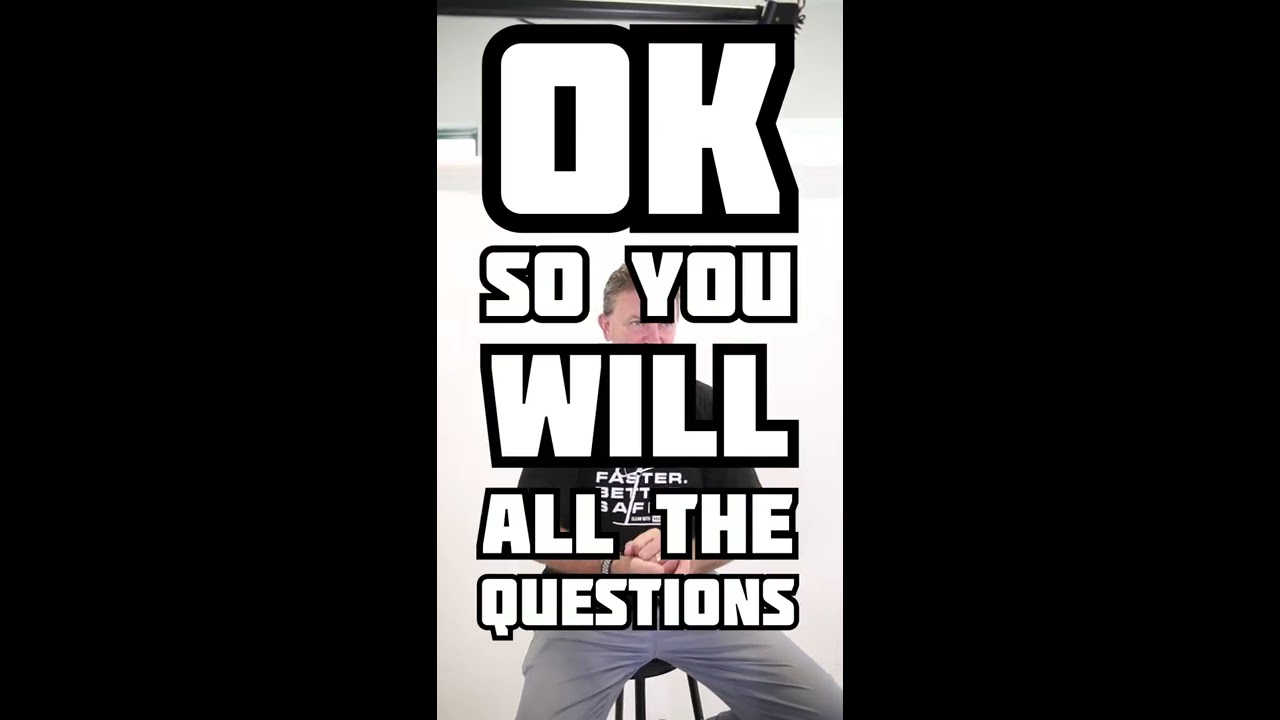The image is a stylized photograph divided into three vertical panels, with the left and right panels being entirely black. The center panel features a man sitting on a stool against a ambiguous white background, which could be a wall or curtain. This man, who bears a resemblance to actor Jeremy Renner, is wearing a black t-shirt with the phrase "Faster, Better, Safer" partially visible and gray cargo pants. He appears to have short light brown hair, white skin with reddish cheeks, and his hands are resting together in front of his stomach. Overlaid on the photograph is a gradient of text that starts large at the top and progressively gets smaller as it descends. The text, in bold white lettering outlined with black, reads: "Okay, so you will all the questions." This thoughtful composition gives a clear focus to the central figure while the black panels create a framing effect that highlights the text and the subject.